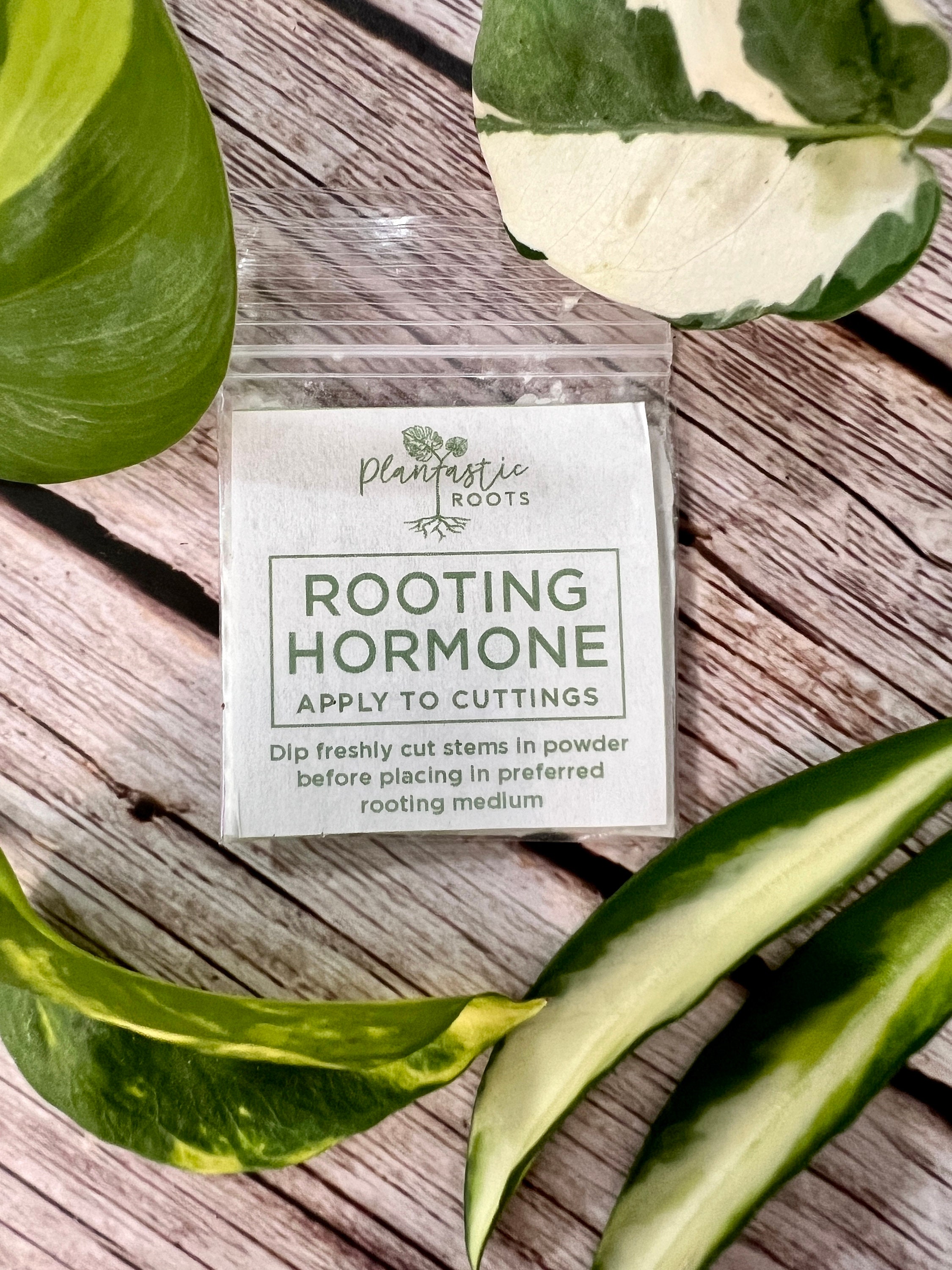This photograph serves as an advertisement featuring various types of plant leaves arranged artistically around a Ziploc bag containing rooting hormone. The bag prominently displays the logo "Plantastic Roots" with instructions that read, "Apply to cuttings, dip freshly cut stems in powder before placing in preferred rooting medium." The leaves, which appear to be healthy cuttings from different indoor plants, encircle the Ziploc bag, all laid out on a heavily weathered, unpainted, gray wooden surface—suggestive of an old wooden table or bench. The grayed, distressed wood makes for a very attractive and rustic background. The arrangement vividly highlights the rooting hormone product, presumably enhancing the speed and success of plant transplantation.